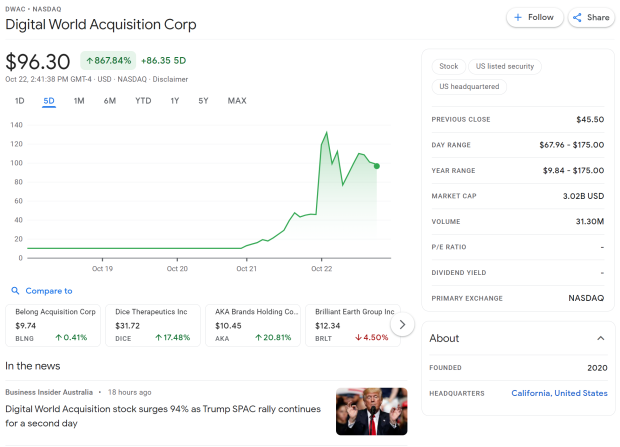**Detailed Caption:**

The screenshot prominently displays stock information for DWAC on NASDAQ. At the upper left corner, it clearly shows "DWAC NASDAQ" with "Digital World Acquisition Corp" written underneath. On the far right, there are interactive buttons labeled "Follow" and "Share." Below this, the stock price is listed as $96.30, accompanied by a significant increase indicator, "867.84%" with an upward-pointing arrow. Underneath, the date and time are marked as "October 22, 2:41:38 PM GMT-4 USD."

The image features a graph charting the stock's performance from October 19 to October 22. Below the graph, there's a "Compare to" option with additional charts available for comparison. In the news section, an article headline from Business Insider Australia highlights that "Digital World Acquisition stock surges 94% as Trump SPAC rally continues for a second day."

On the right side of the image, there is detailed stock information, including the previous close, day range, year range, market cap, and volume, providing a comprehensive overview of the stock's performance and metrics.